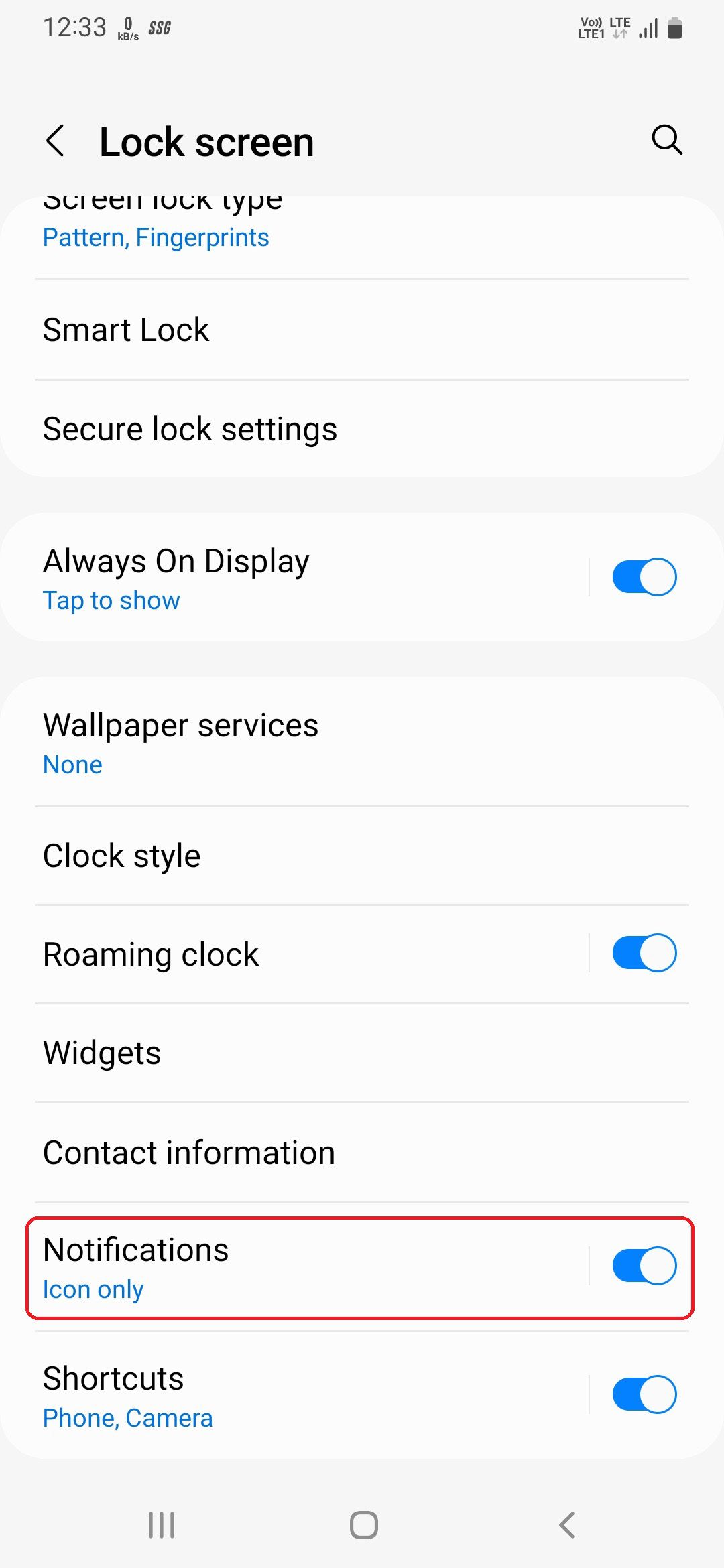This screen capture shows the lock screen settings of a smartphone at 2:33 PM with an 80% battery charge and full network signal bars. The lock screen configuration details are as follows:

- **Screen Lock Type**: Pattern, with an alternative option for fingerprints.
- **Smart Lock**: Enabled.
- **Secure Lock Settings**: Configured but not detailed in the image.
- **Always On Display**: Activated, with the "Tap to Show" option highlighted in blue.
- **Wallpaper Services**: None selected, using the original setting.
- **Clock Style**: Roaming clock feature activated.
- **Widgets**: No widgets listed.
- **Contact Information**: Not provided.
- **Notifications**: Set to "Icon only," and this feature is turned on.
- **Shortcuts**: Quick access to phone and camera is enabled.

This detailed overview summarizes the current lock screen settings, highlighting active features and areas lacking customization.